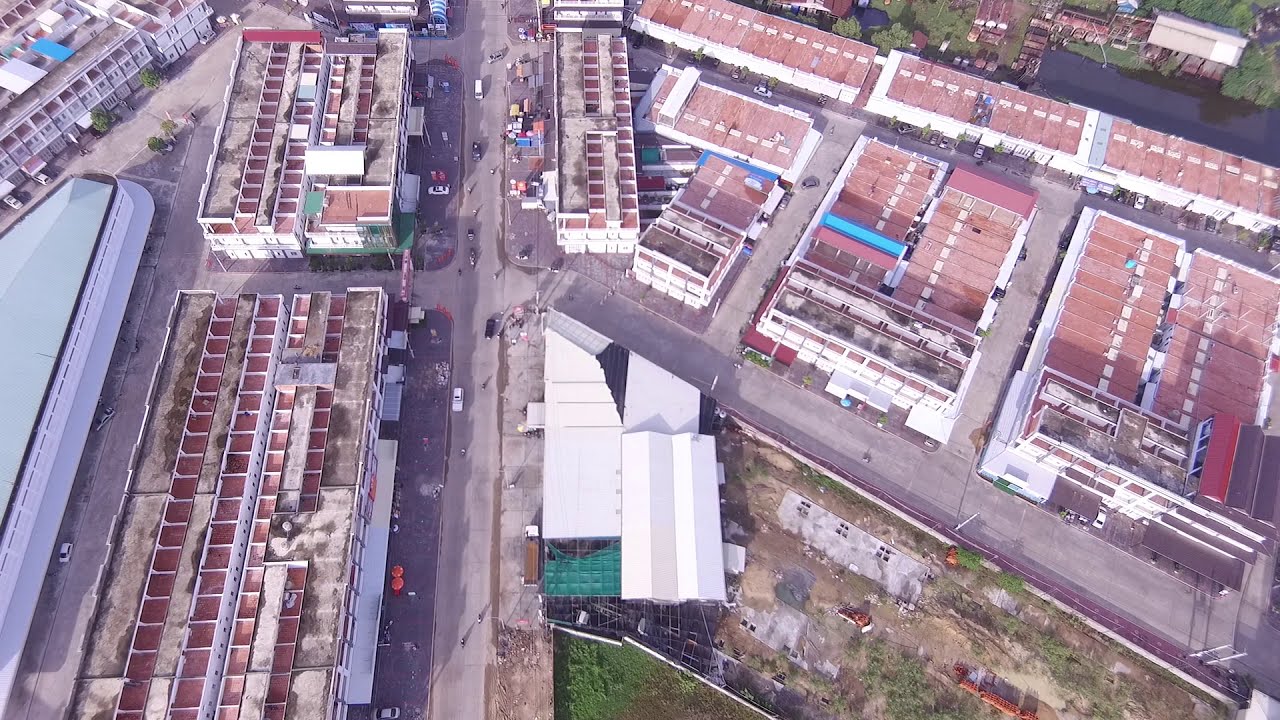The image is an aerial photograph taken from a high vantage point, likely by a drone or a helicopter, capturing a detailed view of an industrial area or business district. Dominating the scene is a main road running north to south, situated approximately 40% from the left edge of the image. This road is populated with moving cars and vehicles parked on both sides. The composition also includes multiple streets, with two parallel ones on the left side extending from the top to the bottom, and a central street connecting them. Additionally, two perpendicular streets branch out from the main road to the right side of the image.

The area is characterized by a grid of industrial buildings with flat, rusted, or lightly colored rooftops, and some roofs displaying shingles. The structures are multi-storied, with flat sides possibly made of brick or cinder block, fitting a stereotypical industrial appearance. In terms of greenery, the landscape is quite barren, with minimal foliage—only a small patch of green visible in the upper right-hand corner and a bit more at the very bottom center. Daylight illuminates the entire scene, casting clear shadows and highlighting the sparse, concrete-dominated terrain. The overwhelming impression is one of a weathered, possibly impoverished area, devoid of significant vegetation but bustling with vehicular and pedestrian activity.